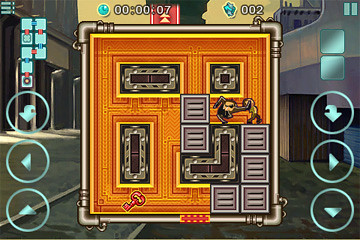The image appears to be a color screenshot from a video game. It is rectangular in shape, slightly wider than it is tall, and features a computer-generated scene. At the center of the image is a prominent orange square with a thin yellow border. Surrounding the yellow border is a layer of silver piping that frames the entire square. Inside the orange square, one can see additional yellow lines, borders, and various small components.

Towards the mid-right of the image, there is a small animated character, suggesting some form of in-game avatar or protagonist. Adjacent to this character are several gray squares stacked vertically, possibly representing in-game structures or objects. The backdrop of the image portrays a dark cityscape, providing a moody, atmospheric setting. On both sides of the image, there are circular elements that resemble button controls, indicating interactive features of the game. Across the top of the screen, status symbols are displayed, likely conveying vital information such as health, score, or inventory status.